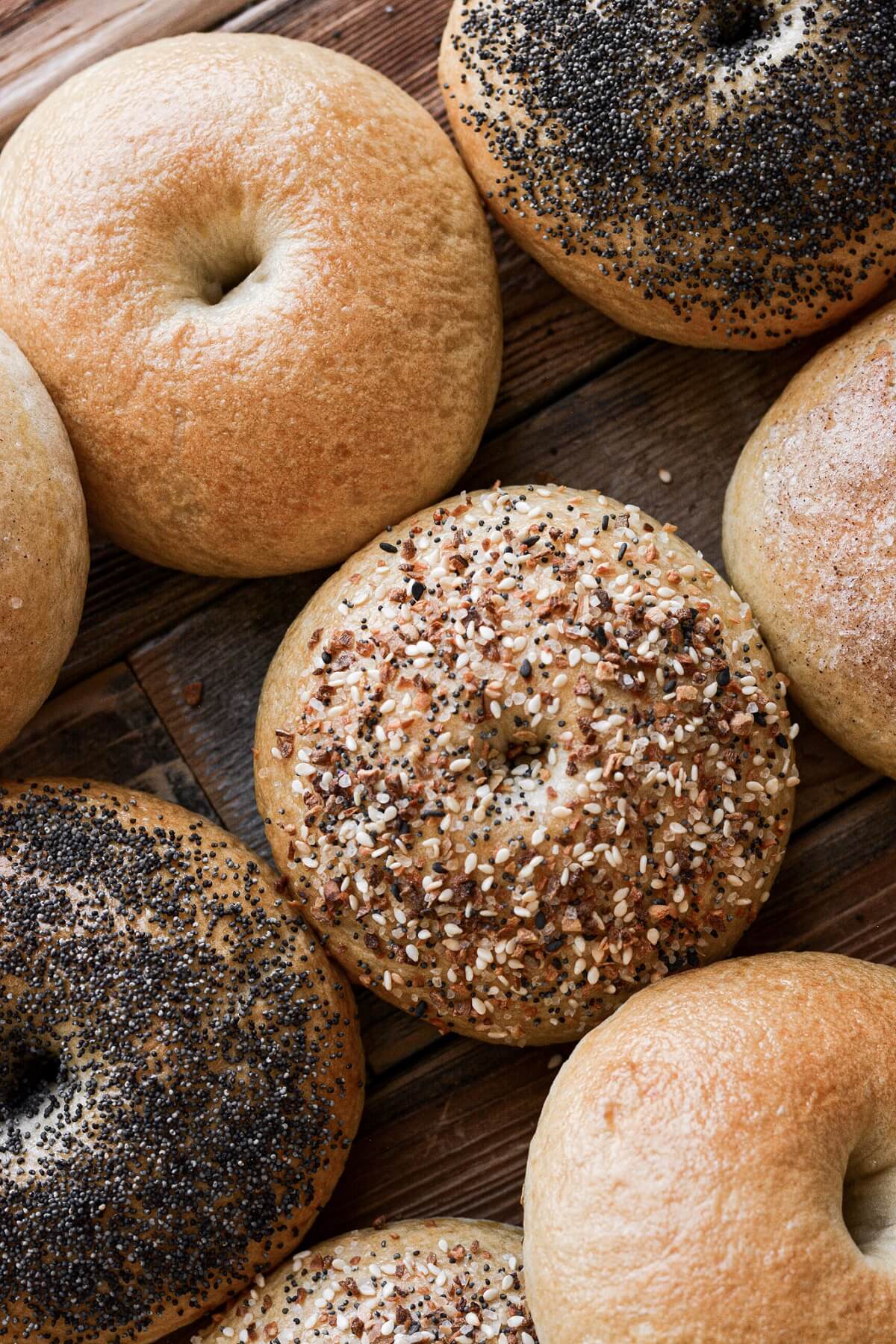This is an overhead photograph capturing a rustic, weathered dark wood table, partially visible between a scattered arrangement of eight bagels. The bagels are placed diagonally from the bottom left to the top right, with three grouped in the top left, three across the middle, and two in the bottom right. The focus is on their varied toppings: a mix of plain, sesame seed, poppy seed, and everything bagels. The plain bagels, tan and light brown in color, contrast with the seeded ones speckled with tiny black seeds and mixed seeds. The holes are small, barely noticeable, creating a puffy, doughnut-like appearance. The rustic table’s brown and black grains provide a natural backdrop for the array of baked goods. The photo, taken from an above angle, emphasizes the texture and arrangement of this collection of bagels against the earthy wooden surface.